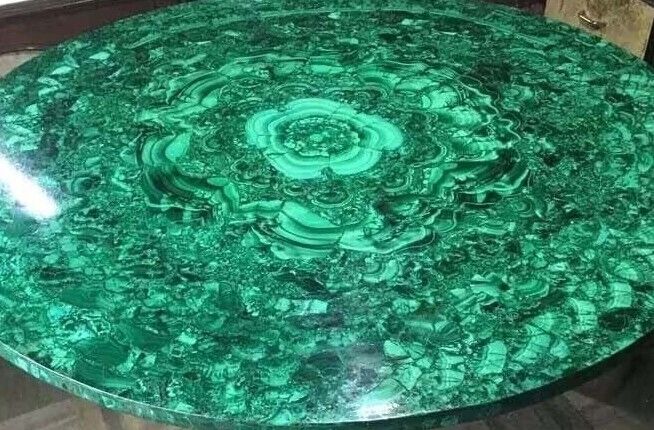The image shows what appears to be a large, marble-like table with a striking emerald green surface. The table's top is dominated by a rich green color with intricate, swirling patterns, which include various shades of green ranging from dark to light, and what some describe as white specks. These patterns radiate outward from the center, reminiscent of tree rings, creating a visually captivating design. The surface has a noticeable sheen, with harsh glints of reflected light on the left side and the bottom, adding to its glossy, marble-like appearance. The backdrop of the image includes a gray and white carpet at the lower edge and a drawer in the back right corner, suggesting the setting is a room, although the table's legs are not visible. The overall impression is one of a stunning, ocean-green table with elaborate and detailed marbling patterns, set against a modest floor background.